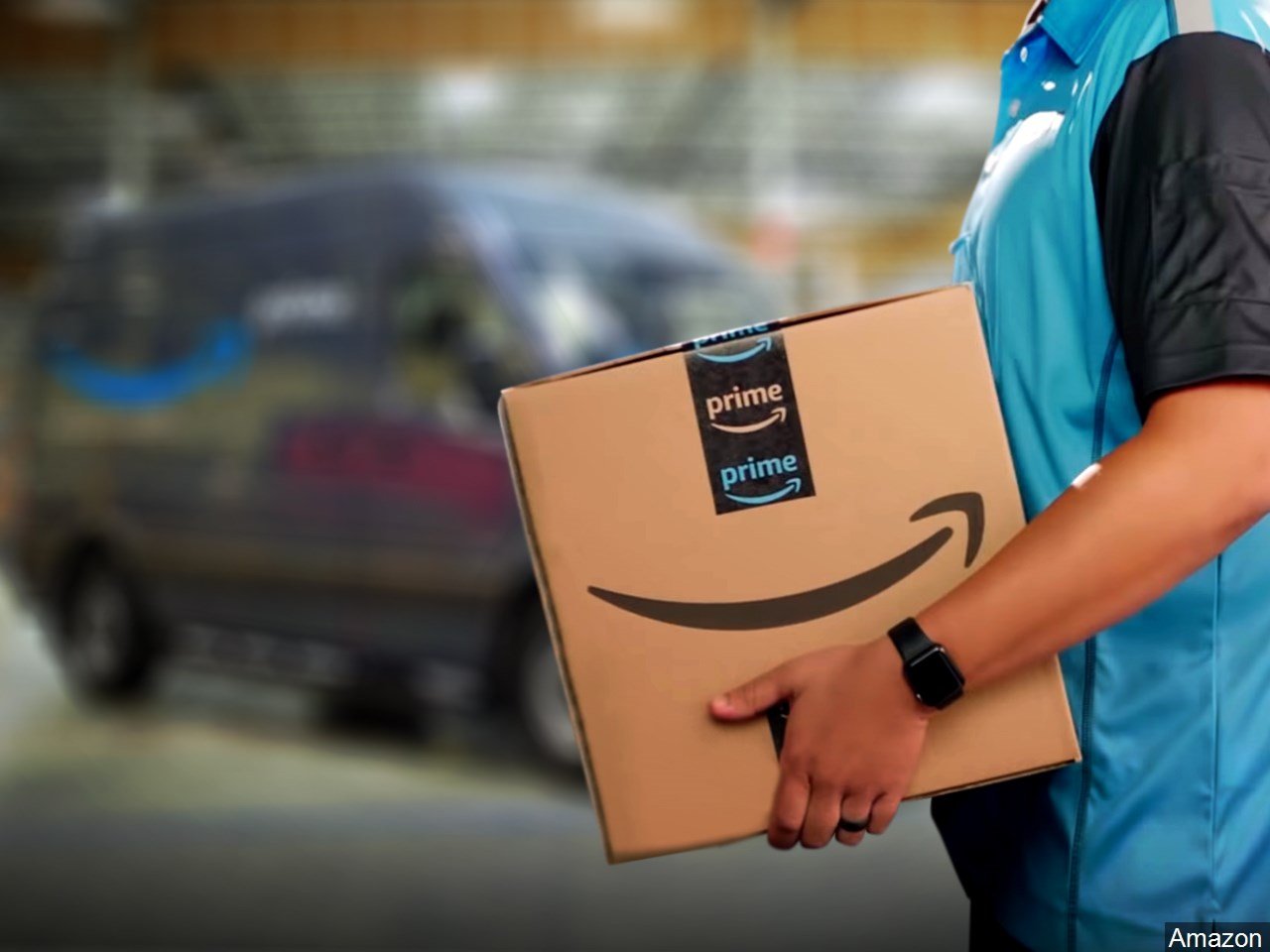In this image associated with Amazon, a medium-complexioned Amazon worker is prominently featured in the foreground. The worker is wearing a standard-issue Amazon shirt, characterized by its blue body, black shoulder sleeves, a gray stripe along the shoulders, and a button collar. A black wristwatch adorns their wrist. The worker is holding a medium-sized Amazon box, easily identifiable by the Amazon insignia and the distinct Prime tape sealing it. The background, slightly out of focus, reveals a blurry figure of an Amazon delivery truck, suggesting the setting is within a warehouse environment. At the very bottom right corner of the image, the word "Amazon" is displayed in white letters against a navy backdrop.